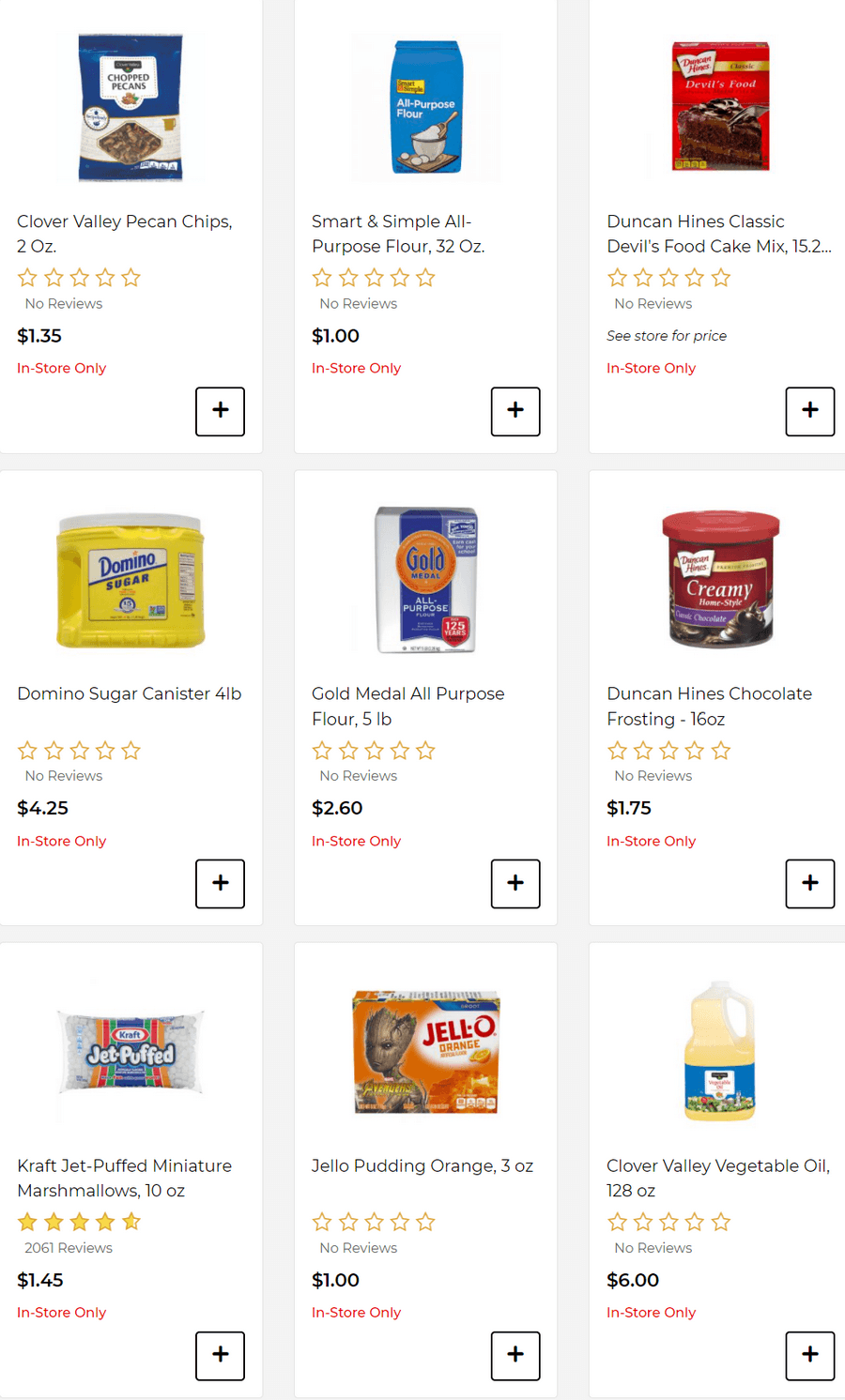The image depicts an online grocery store webpage displaying nine items available for in-store purchase only. All items are marked with "no reviews" and a bold red "in-store only" label, while the remaining text, including product names and prices, is in black. The products shown include:

1. Clover Valley Pecan Chips
2. Smart and Simple All-Purpose Flour
3. Duncan Hines Classic Devil's Food Cake Mix
4. Domino Sugar Canister
5. Duncan Hines Chocolate Frosting
6. Kraft Jet-Puffed Miniature Marshmallows
7. Jell-O Orange Pudding
8. Clover Valley Vegetable Oil

Each item is accompanied by detailed weight information listed in either ounces or pounds. The pricing for the items ranges between $1 to $6.